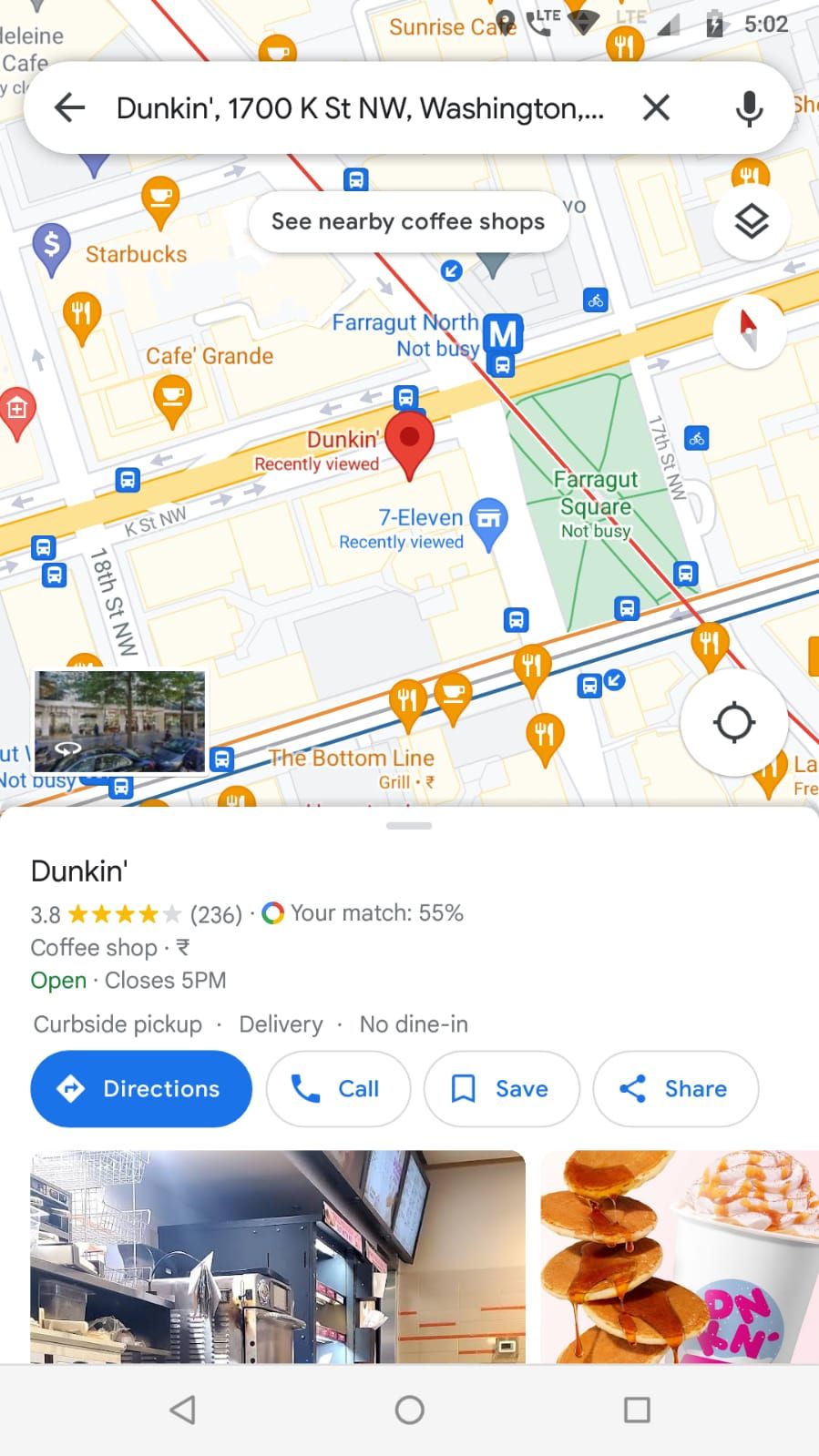This image is a screenshot of a detailed map interface, occupying most of the webpage. At the top, there is a search bar with a left-pointing arrow, displaying the address "Duncan, 1700 K Street, Northwest Washington." Below the search bar, there is a prompt that says "See nearby coffee shops," followed by streets, locations, and other landmarks visible on the map to provide geographic context within the actual city.

The specific location for "Duncan" is highlighted, indicating it has a rating of 3.8 stars from 236 reviews, with a match percentage of 55% for the user. It is identified as a coffee shop that operates until 5 PM, offering curbside pickup and delivery services, but no dining options. 

Further options are available for the user: a blue-colored ‘Directions’ tab, and white-background tabs with blue text for 'Call,' 'Save,' and 'Share.'

Beneath these details, there are two images: one on the left showing the interior of Duncan with a kitchen, a coffee maker, and a menu board. The image on the right depicts a plate of pancakes drizzled with syrup, alongside a drink topped with foam and caramel.